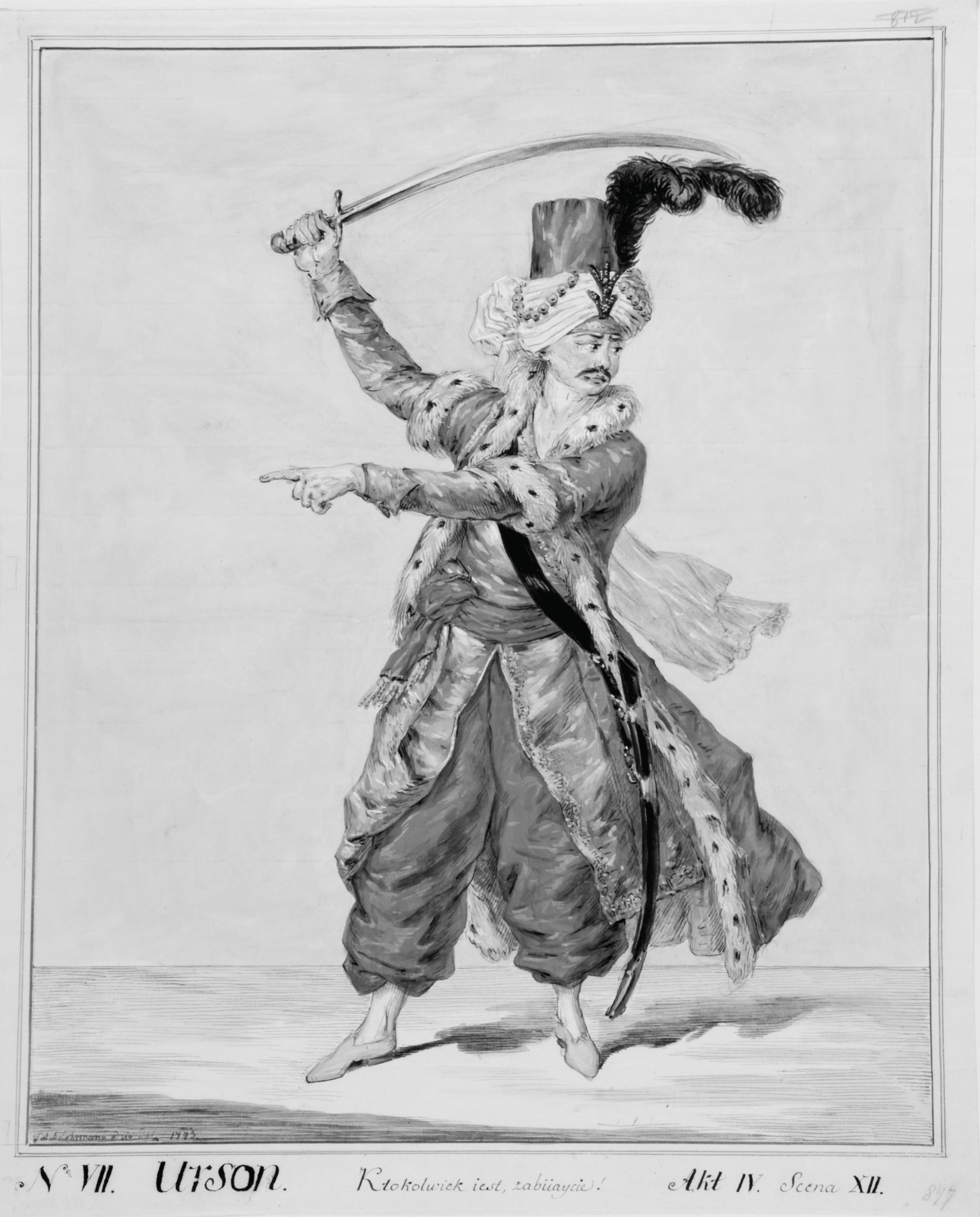This is a highly detailed black and white illustration resembling a poster, depicting a warrior dressed in elaborate, ancient attire reminiscent of an Arabian Nights or possibly Ottoman Empire figure. He is adorned with a turban, complemented by a top hat and elaborate feather plumes curling outwards. The warrior wears a fur-lined robe or cape that extends to his ankles, featuring fur around the collar and cuffs. Underneath, he dons wide, puffed pantaloon-style pants tucked into slippers. His attire includes a tuxedo-like shirt, and he has a flowy scarf draped around him. A cross-body sword sheath is visible, carrying a long, curved scimitar which he brandishes overhead with one hand, while his other arm points across his body towards the left. The image has some text in an unidentifiable language, adding to the historical and exotic atmosphere of the illustration.